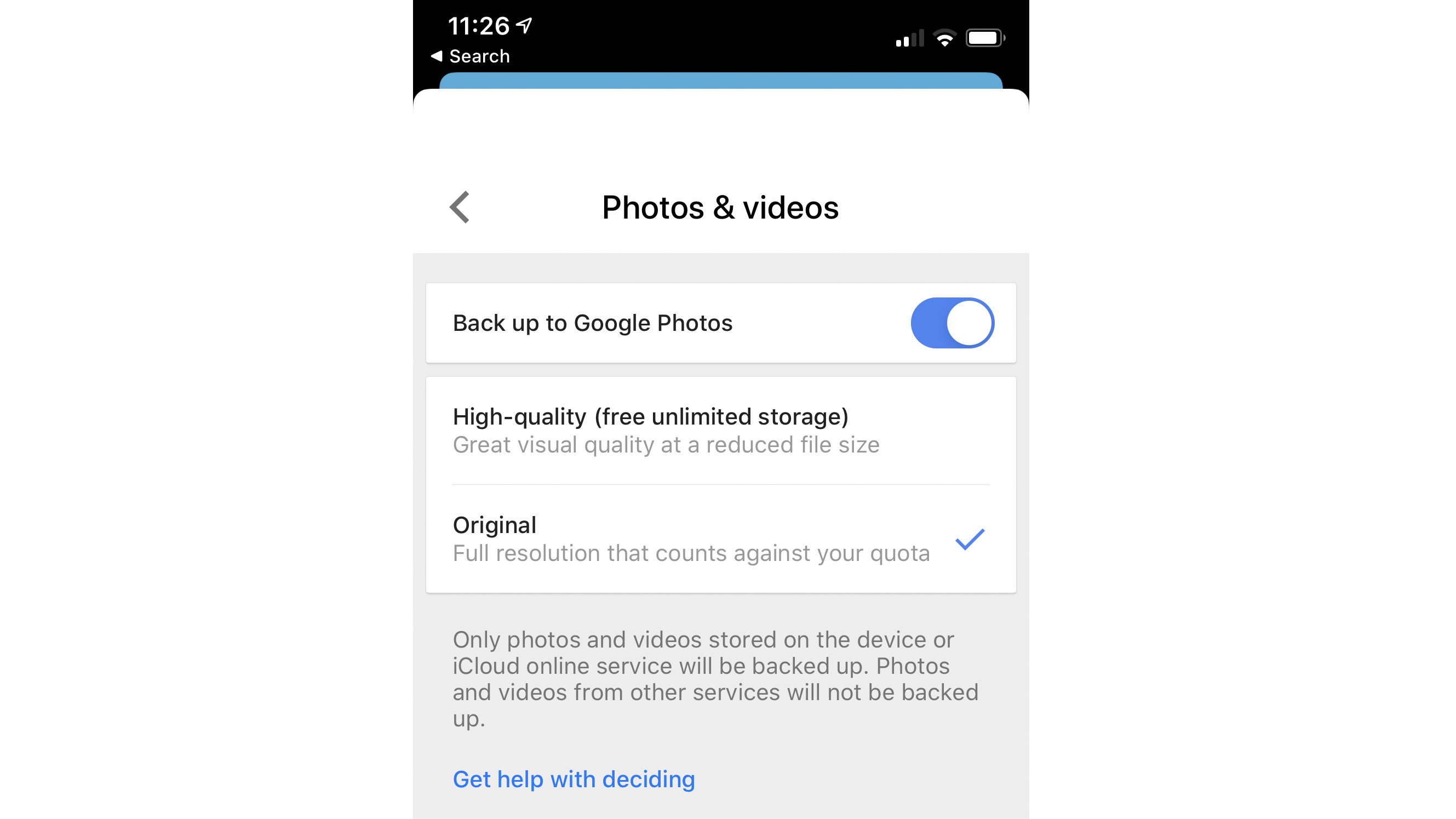The screenshot features a smartphone settings page dedicated to "Photos and Videos" centered on a white background. At the top, there is a black header displaying the current time in white text, a search link below it, and network connectivity icons along with a nearly full battery icon on the right. Beneath this is a thin sky-blue bar that separates the header from the main content.

The main page is titled "Photos and Videos." Directly below this header is a banner labeled "Backup to Google Photos," accompanied by a blue active toggle switch. Following this is another banner entitled "High Quality" with the note "(Free Unlimited Storage)" and a brief line of content information below it.

Next, the section labeled "Original" appears, paired with a line of information and a small blue check mark. Further down the page, there's a paragraph detailing the application's settings. At the bottom, a help section features blue text that reads "Get Help with Deciding."